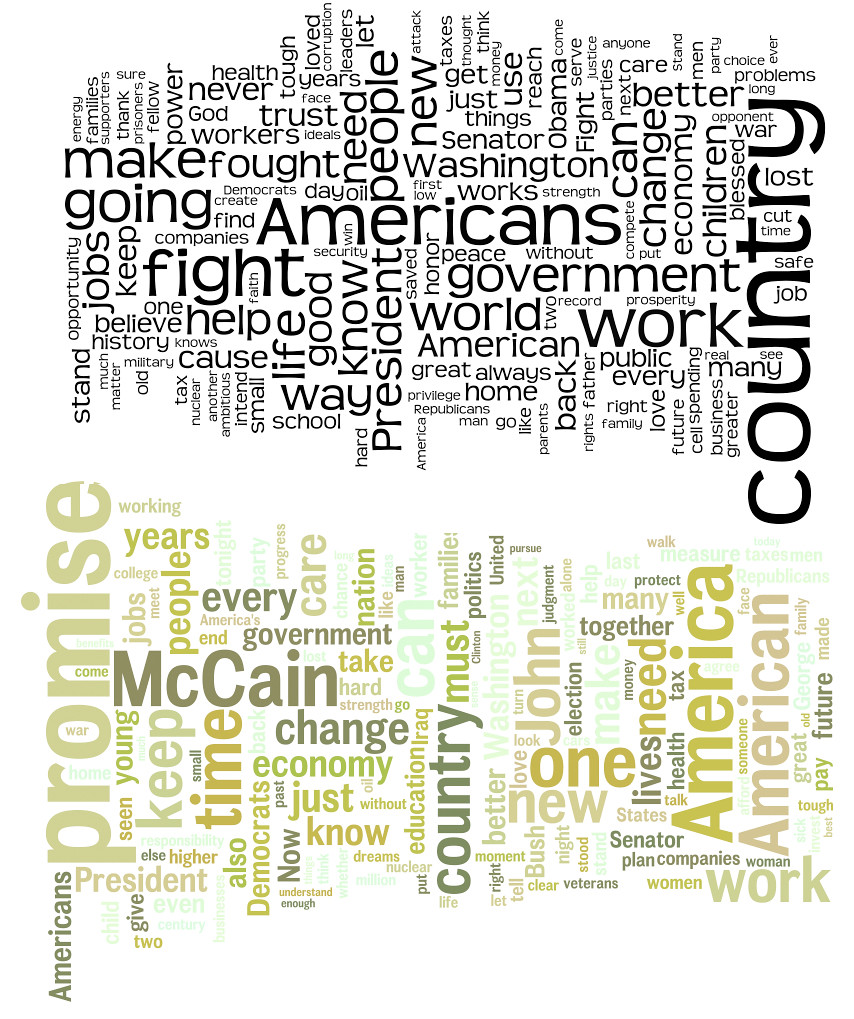The image is a political poster with a distinctive white background and presents a word collage, designed in a puzzle-like arrangement. The top half predominantly features words in black, with a few larger, bold black words such as "Americans," "country," and "fight." Surrounding these are smaller words like "government," "work," "make," "Senator," "Washington," "peace," "always," and "home." A thin white dividing line splits the composition, below which phrases appear in varying shades of green, including khaki and light green. Notable words in this section include "America," "American," "McCain," "change," "every," "government," and "one." Additionally, the left-hand side features the word "promise" in paler green. The poster emphasizes a political message through its organized yet crowded arrangement of impactful words.